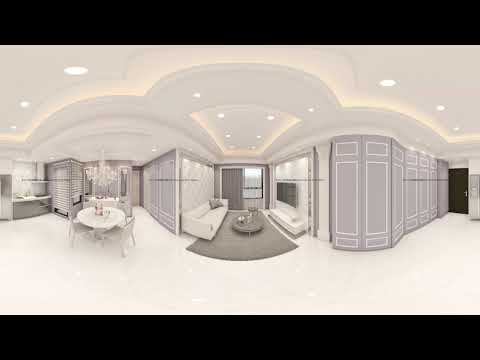The image presents an all-white, monochromatic space that creates an illusion of a black and white reality by combining only shades of white, gray, and some black elements. The room is divided into two segments. On the left, there is a dining area featuring a white table surrounded by chairs and highlighted by a chandelier above. To the right of the dining area is a living room setup with a large gray rectangular rug, centered with a round table. This area consists of two white couches—a sofa on the left and a loveseat on the right—positioned around a fireplace, which anchors the back of the room. A gray curtain adorns the window behind the living room setup. Paneled walls with rectangular designs and a dark-colored door occupy the right-hand side of the image. The entire composition, including the furniture and décor, is predominantly white with subtle variations of light gray, creating a striking, coherent monochrome aesthetic. The framing of the image and certain architectural details, like the arched figure and framed edge, evoke a sense of depth and illusion, making the space appear both cohesive and segmented at the same time.